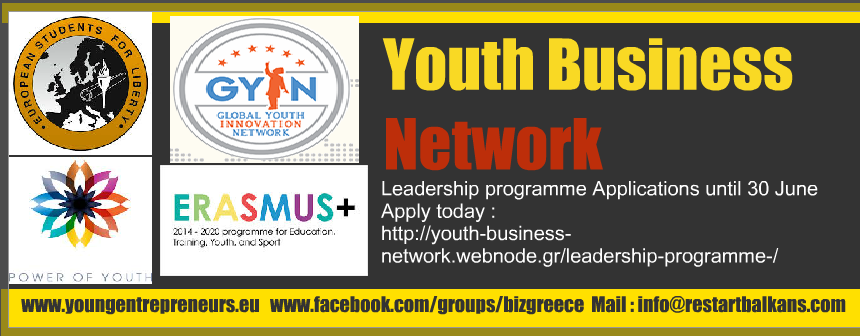The image is a long horizontal advertisement banner with a black background and yellow and red text. The main heading reads "Youth Business Network" in yellow and "Network" in red. On the left side, there are various sponsor logos including a rainbow-colored flower logo with "Power of Youth," another reading "George Youth Innovation Network," and others such as "Global Youth Innovation Network," "Erasmus," and "European Students for Liberty." The banner announces, "Leadership Program Applications until June 30th. Apply today!" Below this are several web addresses: "youthbusinessnetwork.webnode.gr/leadershipprogram," "www.youngentrepreneurs.eu," and "www.facebook.com/group/bizgrease." Additionally, an email address is provided: "mail info at restartbalkans.com." The overall design is reminiscent of an internet graphic, possibly used as a website banner.